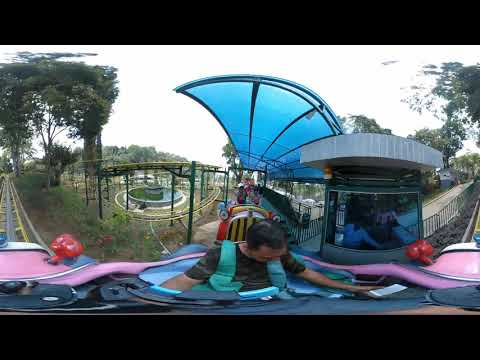In this distorted fisheye photograph, a man with black hair, slightly tilting his head downward to the right, is seen on a roller coaster ride at an amusement park. He is wearing a dark green shirt with light green straps over his shoulders, which give the appearance of a harness. His right arm is extended to the side, holding a stretched white piece of paper due to the lens distortion. The pink-colored cart of the roller coaster frames him, with the yellow and gray track visible on both sides. Above him is a light blue canopy with black support lines. To the right of this canopy, a building with a gray roof and lined undersides houses a large screen displaying images. Further to the right, a black barrier extends into the background. In the center-left section of the image, there appears to be a round fountain with green water and a structure propped on green poles. Tall green trees dot both sides of the picture, and the sky above is a solid, hazy white, contributing to the overcast ambiance.